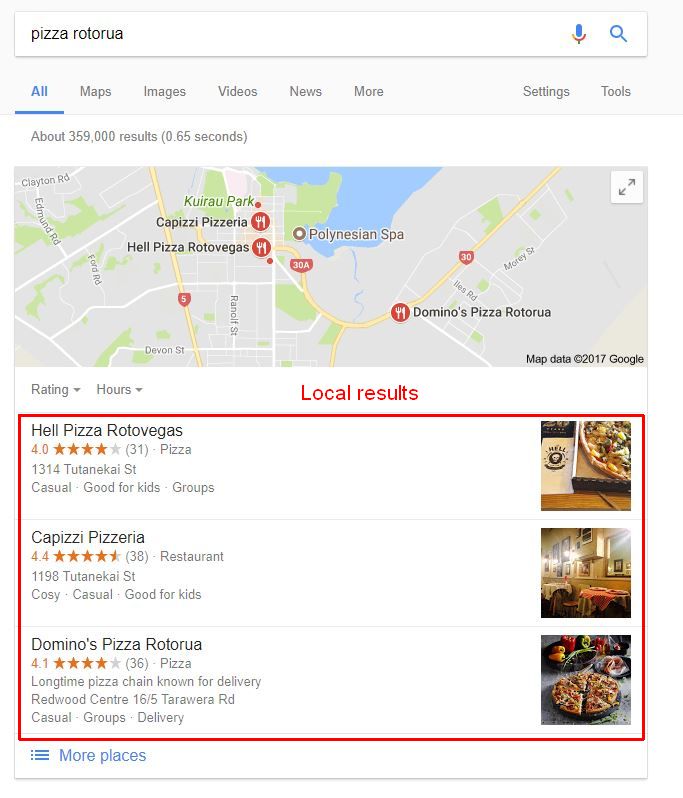This image depicts an advertisement for various pizza restaurants, prominently featuring the search term "Pizza Ratora" within a search bar at the top. The search bar includes an icon of a microphone and a magnifying glass to the right. Below this, the interface displays several tabs labeled "All," "Max," "Images," "Videos," "News," "More," with "Settings" and "Tools" appearing slightly separated but on the same line. The results indicate approximately 359,000 matches found in 0.65 seconds.

Beneath this summary, a highlighted rectangular box presents detailed information about various local pizza establishments. Each listing includes fork and knife icons. The first restaurant, "Hell Pizza Roto Vegas," boasts a rating of four stars and highlights its suitability for kids, groups, and casual dining. The address is also displayed. The next listing, "Campisi Pizzeria," garners a 4.4-star rating, features a cozy and casual atmosphere, and is noted as family-friendly. "Domino's Pizza Ratora" also shows a four-star rating, with similar specifics provided about its environment and suitability for children.